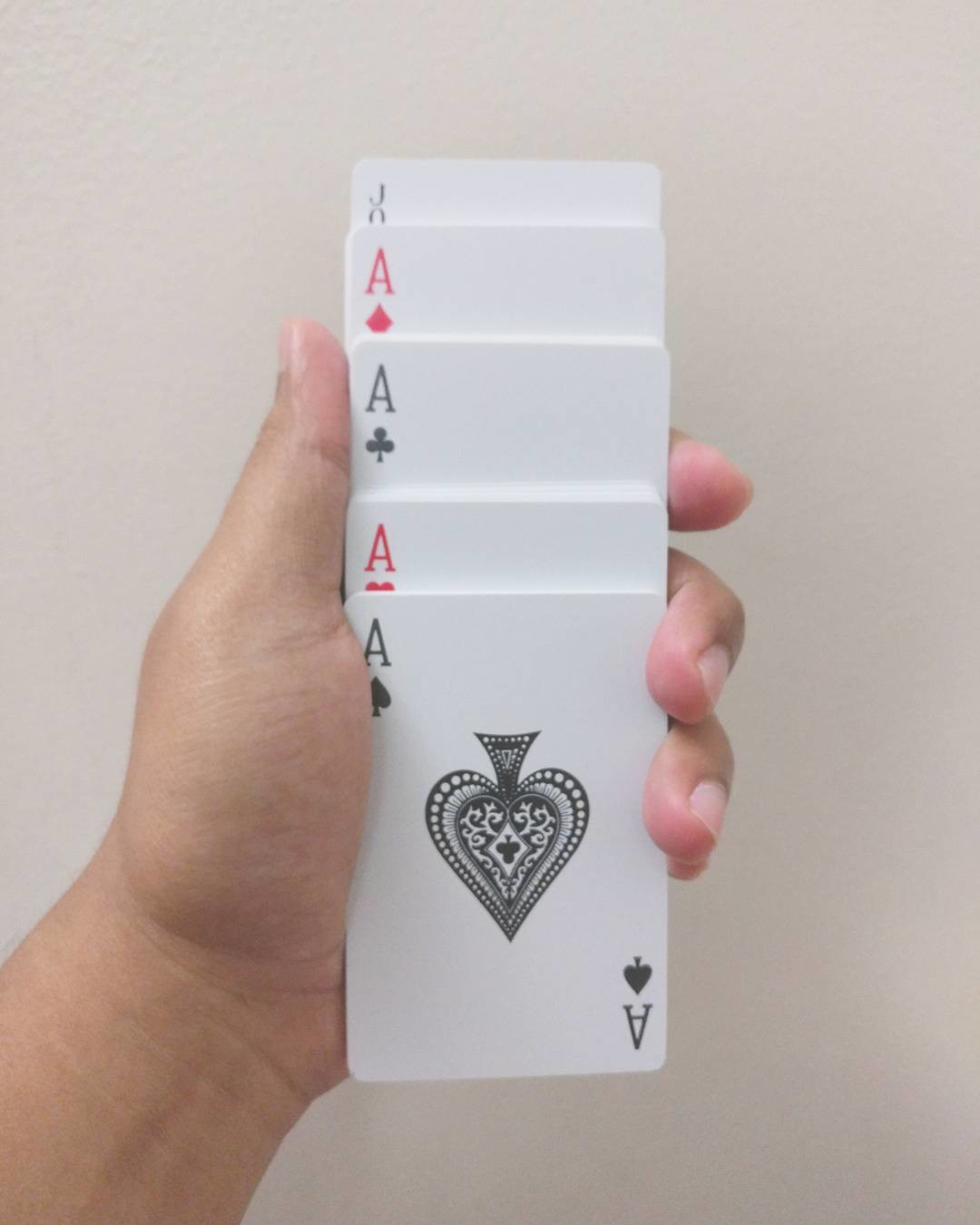In this image, a Caucasian hand with trimmed nails, pink at the tips, protrudes diagonally from the lower left corner towards the center, holding a stack of playing cards. The background is a plain, slightly blurred whitish-pink wall. The hand is positioned palm-up, showcasing the cards in a sequence that includes four aces: the ace of spades, ace of hearts, ace of clubs, and ace of diamonds, arranged in an alternating black-red pattern. Peeking out at the top of the stack is a joker card, identifiable by the visible "J-O" lettering. The cards are stacked as if prepared for a card game, with the joker card slightly overlapping the aces.